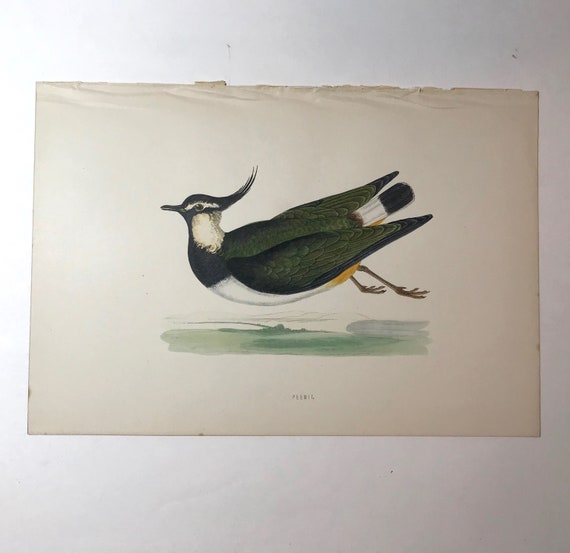The photograph captures a detailed page seemingly removed from a large format book, likely James Audubon's renowned tome on North American birds. The page, frayed on one end, features a meticulously painted bird set against a watercolor background, the artistry executed in either pen or watercolor. The bird, bearing a resemblance to a grouse, is depicted with notable precision and vivid detail. It has dark gray to black feathers with mossy undertones on the wings, transitioning to a black-tipped white tail. The bird's underbelly and the back of its neck are white, while its chest and the front of the neck are black. Distinct upward-sweeping feathers adorn the head, similar in shape to a cardinal's, and a horizontal white streak decorates the area around its eyes, which are black. Its beak is thin and black, contrasting with the bright orange hue of its legs. Additionally, a yellow feather can be noticed near its hind area. Complementing the bird is a green brushstroke representing grass beneath it, enhancing the naturalistic lighting that brightens the left side of the photograph while subtly shadowing the right.